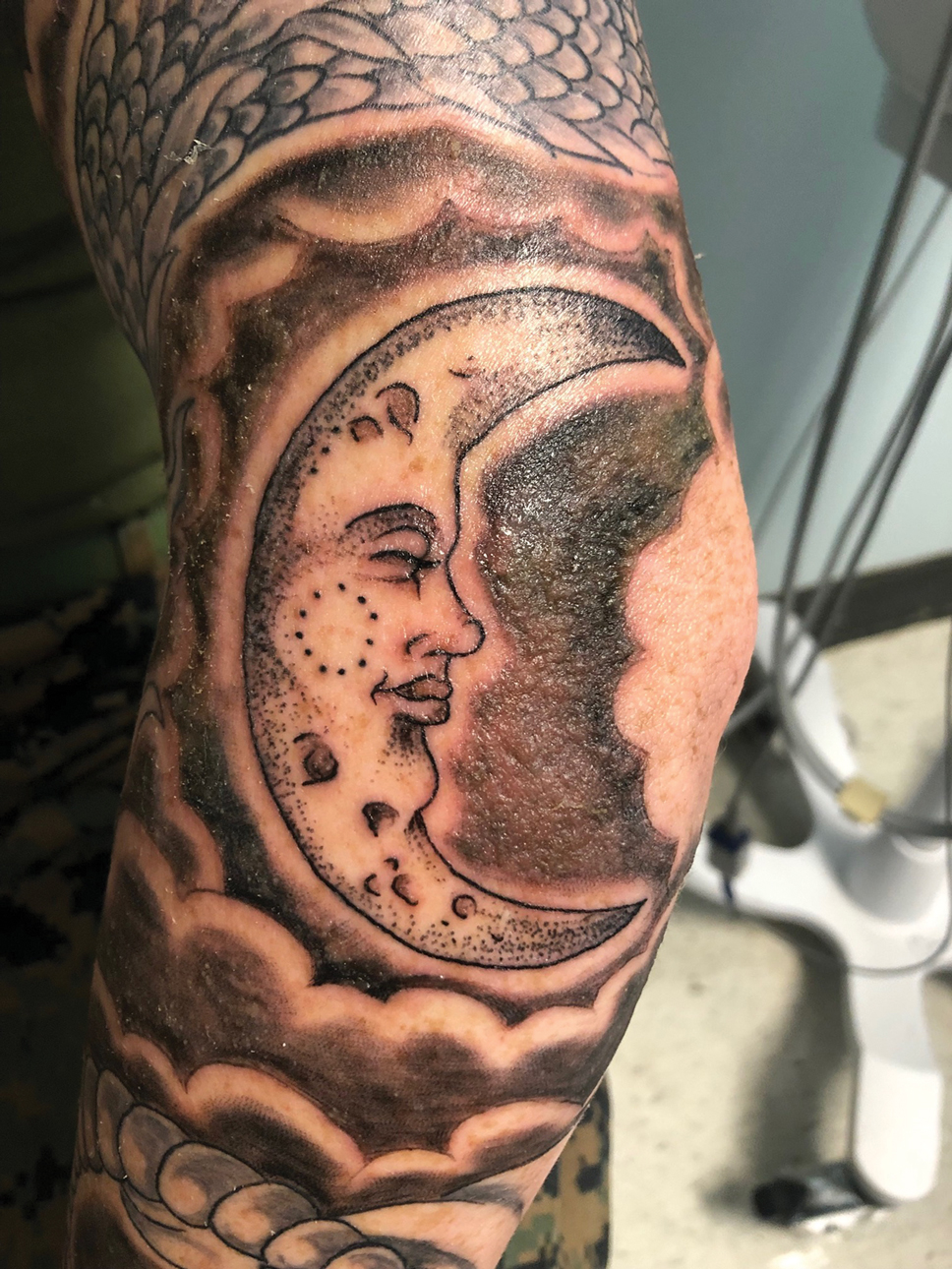The image is a color photograph in portrait orientation, showcasing a detailed view of a tattoo on a person's white and slightly pinkish arm, extending from the shoulder to just below the elbow. The focal point of the tattoo is an anthropomorphic crescent moon with distinct facial features, including lips and a nose that extend beyond the crescent's outline. This blackish-brown tattoo is positioned around the elbow area and is surrounded by dark, fluffy clouds. Above this, a horizontal band featuring a scaly, fish-like design encircles the upper arm. Beneath the crescent moon, a series of bead-like dots accent the tattoo. The background reveals a room interior with a powder blue wall and a white appliance on the right, possibly a stand for a larger appliance, hinting at the setting being a tattoo shop.